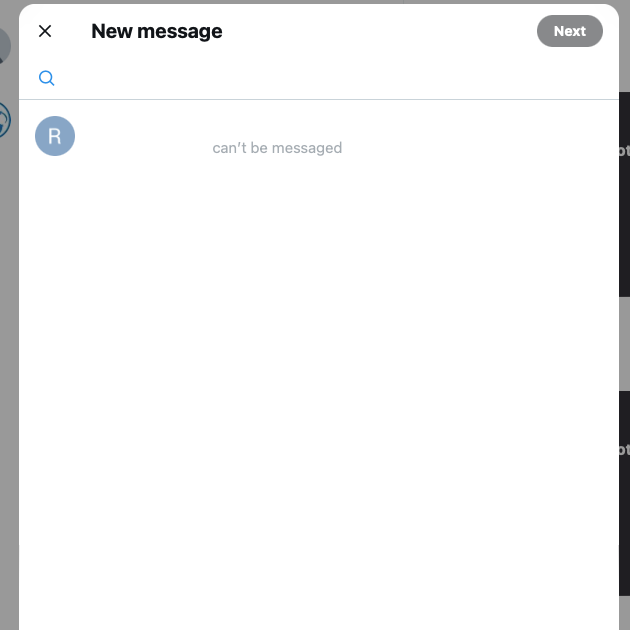The screenshot displays a user interface with a central white rectangle. In the top-right corner of this rectangle is an 'X' icon, indicating the option to close the window. The bold, black text "New message" appears prominently at the top of the rectangle, with "New" capitalized while "message" is in lowercase. Below this title is a gray "Next" button, with its text also capitalized.

Beneath the "Next" button is a blue magnifying glass icon, commonly used to signify a search function. Directly underneath the magnifying glass is a light gray horizontal line stretching from the left to the right edges of the white rectangle. Further down, there is a blue circle with a white 'R' in the center. Adjacent to this circle is the text "can't be messaged," suggesting an unavailable messaging option for this contact.

Partially visible to the right is another screen, barely discernible and cropped off from view. On the far right, there are two black square placeholders, one positioned above the other, hinting at additional content or options outside the main focus of the screenshot.